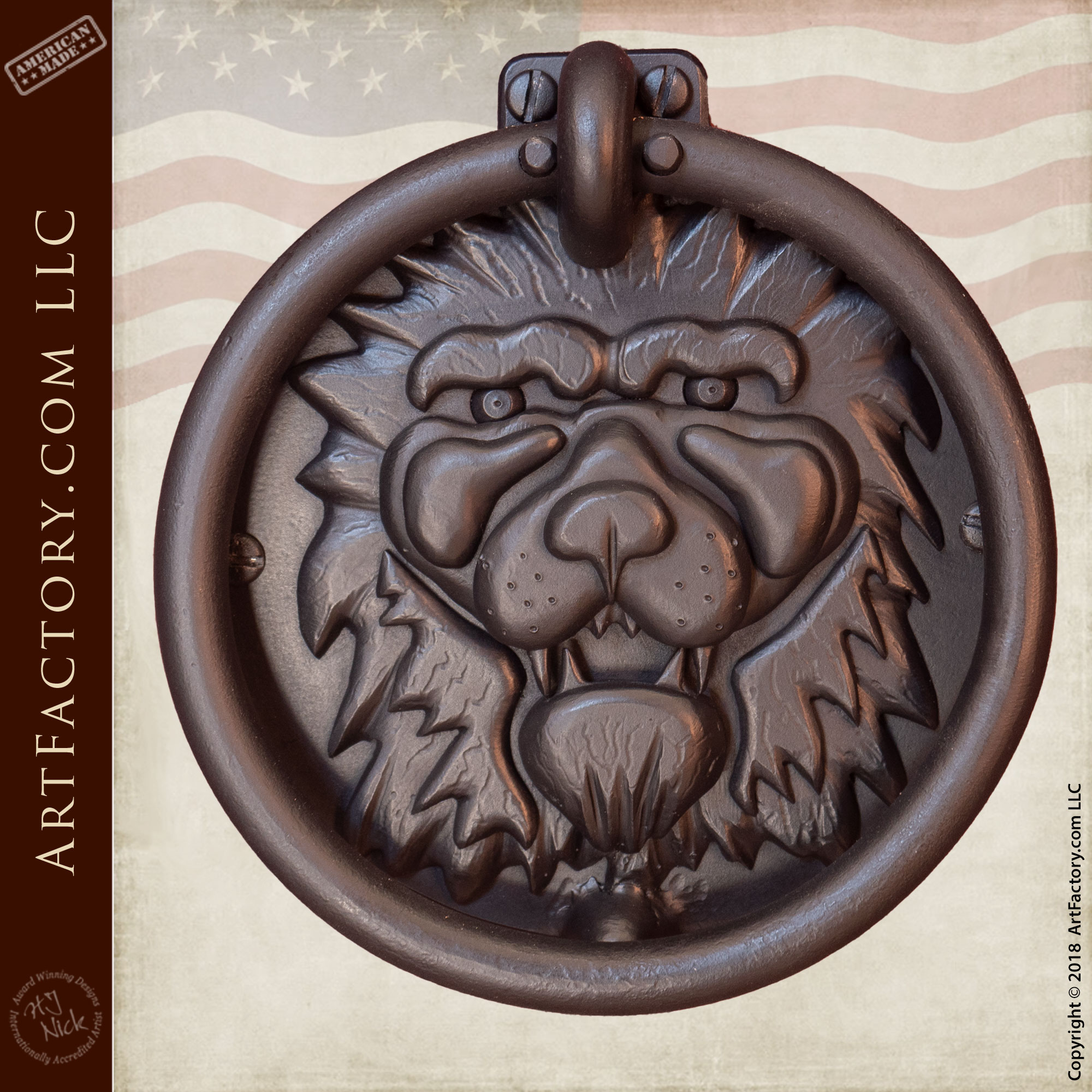The image depicts a detailed metal medallion prominently featuring the embossed, head-on face of a lion with thick eyebrows, prominent cheeks, and thick fur along its jawline, giving it a striking and somewhat abstracted appearance. This medallion has a thick tubular rim and is affixed to a plate with visible screws, suggesting it might function as a decorative door knocker. The entire piece has a chocolaty color and is set against the backdrop of a faded American flag, with three rows of stars visible in the blue field and rippling red and white stripes. At the top left of the image, the text "American Made" is displayed in cream-colored, all-capital letters, angled within a dark strip. Additionally, a circular stamp bearing "H J Nick," along with the copyright mark “2018 ArtFactory.com LLC,” appears at the bottom right. The overall setup and the detailed craftsmanship suggest it is an item for sale from ArtFactory, emphasizing its American heritage.